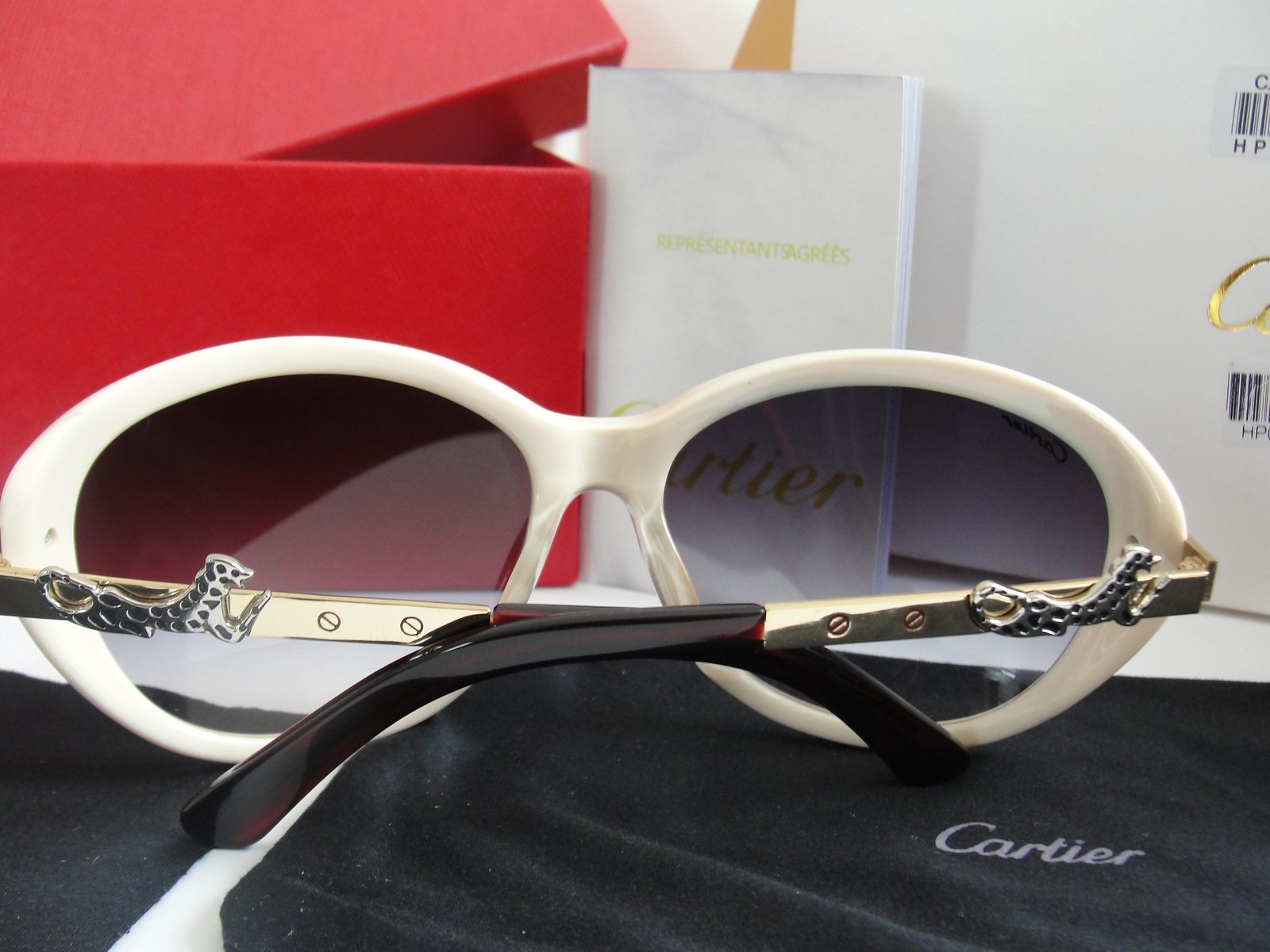The photograph captures a close-up of an exquisite pair of designer sunglasses by Cartier. The ivory-colored, vintage-inspired cat eye frames are presented from behind, emphasizing the elegant arms, which blend a luxurious gold finish with a silver mountain lion or cougar motif on each side. The arms curve into a brownish resin section, designed for comfort behind the ears. The lenses have a subtle gradiated dark tint that adds to their sophisticated appeal. The sunglasses are strategically placed on a piece of black fabric with "Cartier" elegantly inscribed in white, complemented by a partially visible red Cartier box and an open white box in the backdrop. This carefully arranged image resembles what might be shared by an influencer on social media platforms like Instagram, showcasing both the product's opulence and the brand's heritage.